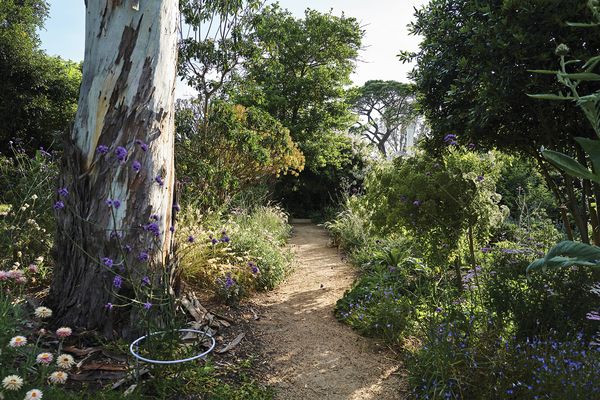The image captures a serene, wild garden-like scene with a dirt walkway, possibly pea gravel, winding through its center. On the left side of the path stands a large tree with weathered white and dark brown bark, surrounded by staked purple columbine flowers, light pink and white wildflowers, and some low brush. On the right side, there's a similar display with additional small purple wildflowers, a large green shrub, and dense undergrowth. The walkway leads towards an entrance enclosed by large trees, offering a glimpse of light blue sky in the distance. Overall, it's a beautifully distinct and naturalistic setting, teeming with vibrant flora beneath a canopy of towering trees.